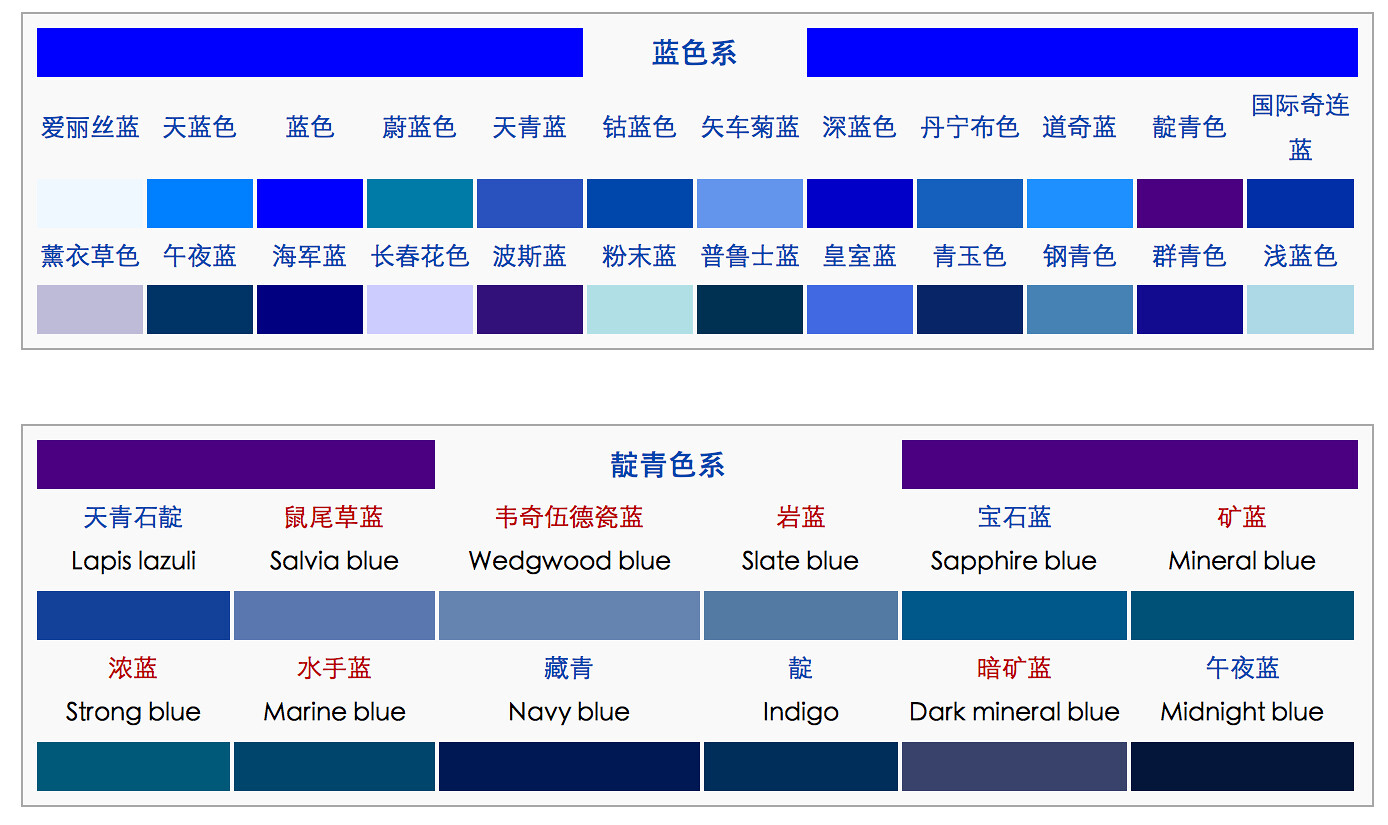The image is a detailed color chart primarily featuring various shades of blue and purple, with text labels in both a foreign language, likely Chinese, and in English. The chart is divided into two main sections:

The top section consists of two long rectangles. The uppermost rectangle is bordered by two vivid blue lines on the right and left sides, with Oriental characters in between. Below this, there is a row of Oriental characters followed by a sequence of side-by-side rectangles in a gradient of blue and purple hues. Another row of Oriental characters appears beneath these colored rectangles, followed by an additional line of same-sized rectangles in various shades of blue, gray, and purple.

The bottom section mirrors the layout but includes English labels. This section is marked by a rectangle flanked by two equal purple lines with Oriental characters in between. Below this, a row of Oriental characters is followed by a row of English color names: "lapis lazuli," "salvia blue," "wedgewood blue," "slate blue," "sapphire blue," and "mineral blue," each paired with a corresponding colored rectangle. Another row of Oriental characters follows, succeeded by another row of English color names: "strong blue," "marine blue," "navy blue," "indigo," "dark mineral blue," and "midnight blue," again each paired with a corresponding colored rectangle.